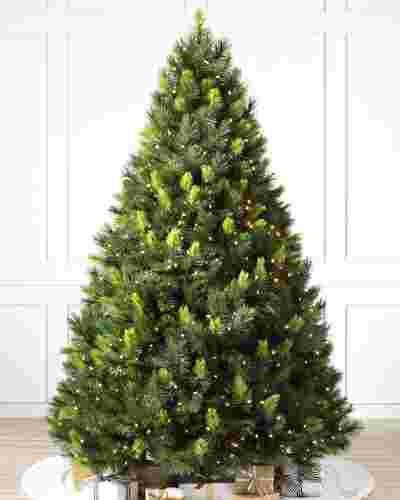The image captures an intricately staged Christmas setting, dominated by a large, triangular-shaped Christmas tree that showcases varying shades of dark and light green. The tree is adorned with an array of small, white LED lights elegantly wrapped around its branches. Beneath the tree, a round cloth carpet with a gold hem accents the light tan wooden floor. Surrounding the base, there are numerous impeccably wrapped presents in neutral tones, suggesting a corporate touch. The backdrop features a heavily pixelated, 3D-looking wall with square trim designs, adding a textured, albeit distorted, element to the setting. The overall composition, centered around the Christmas tree, evokes a festive indoor scene, rich with hues of white, gray, yellow, brown, and green.